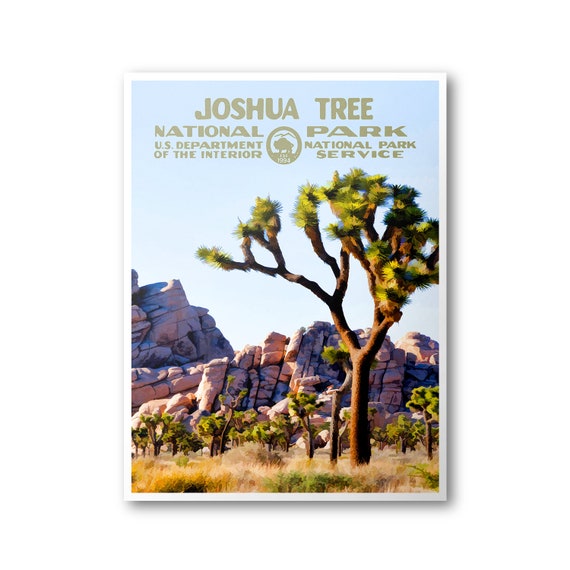The image is a stylized poster set against a white wall, depicting the scenic beauty of Joshua Tree National Park. Dominating the scene is a large, tall tree with a sturdy brown trunk and lush green leaves, standing prominently in the foreground. The tree is rooted in a field dotted with grassy patches and bushes in various shades of beige, yellow, and green. Surrounding this main tree are several smaller trees that add depth to the landscape. In the background, a massive rocky cliff stretches across the image, its highest point reaching towards the left side, and it is studded with larger boulders in a brownish-red hue. The sky is a soft, eggshell blue that provides a serene backdrop for the natural elements. At the top of the poster, in bold golden letters, it reads "Joshua Tree National Park." Below this, it states "U.S. Department of the Interior, National Park Service," accompanied by a circular logo in the center of the text.